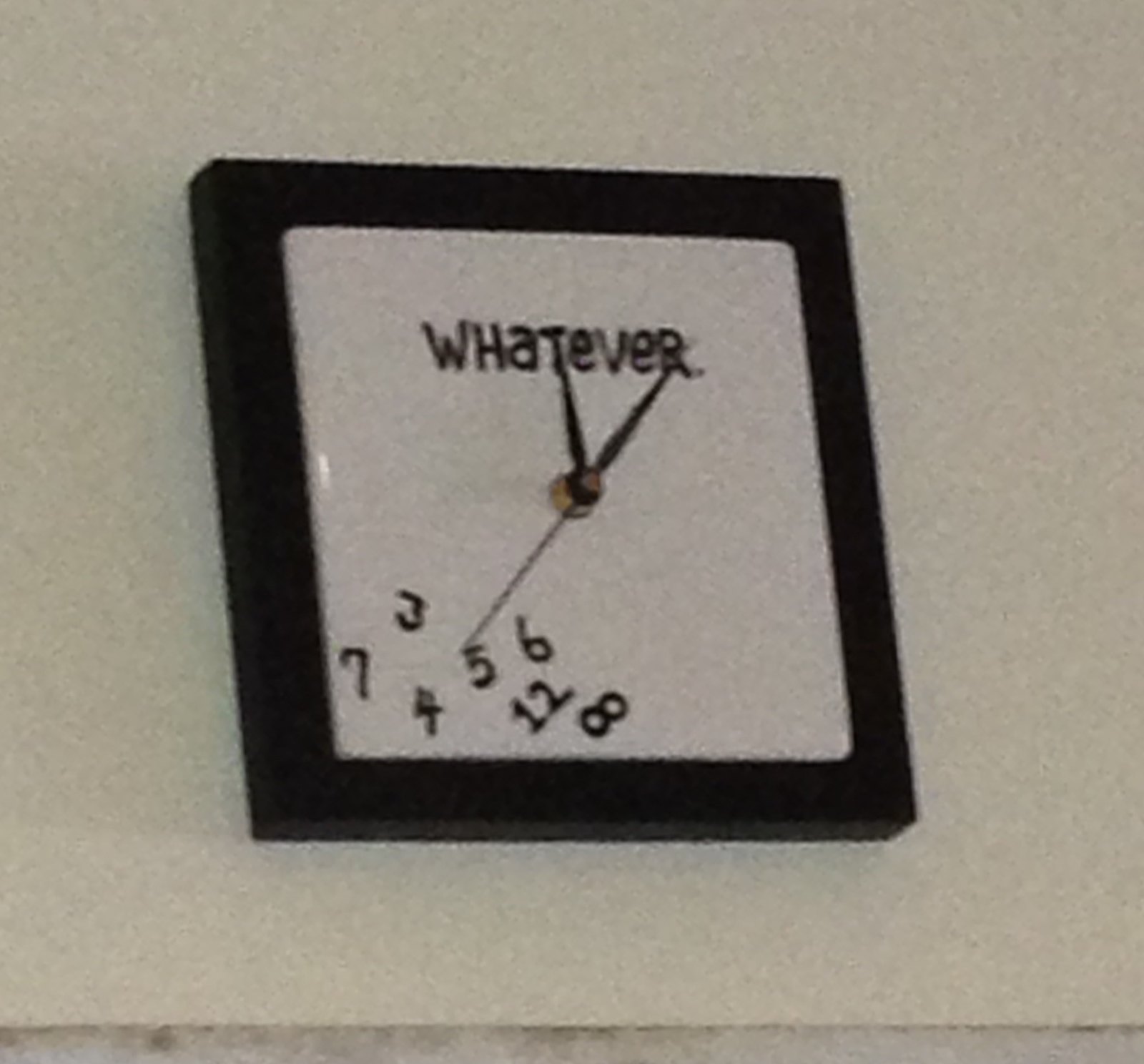This is an illustration of a clock set against a beige wall, creating a warm and neutral background palette. The clock itself stands out with a sleek black trim encasing its circular frame. The interior of the clock face is also beige, seamlessly blending with the backdrop. Prominently displayed at the top of the clock face is the word "Whatever" in a casual, handwritten style. The clock features traditional hour and minute hands in a dark brown hue, complemented by a slender, long second hand in the same dark brown color. Unconventionally, the clock's numbers are scattered at the bottom half of the face, with numbers such as 8, 4, 5, 6, 7, and 3 visible in a quirky, jumbled arrangement, adding a whimsical touch to the overall design.